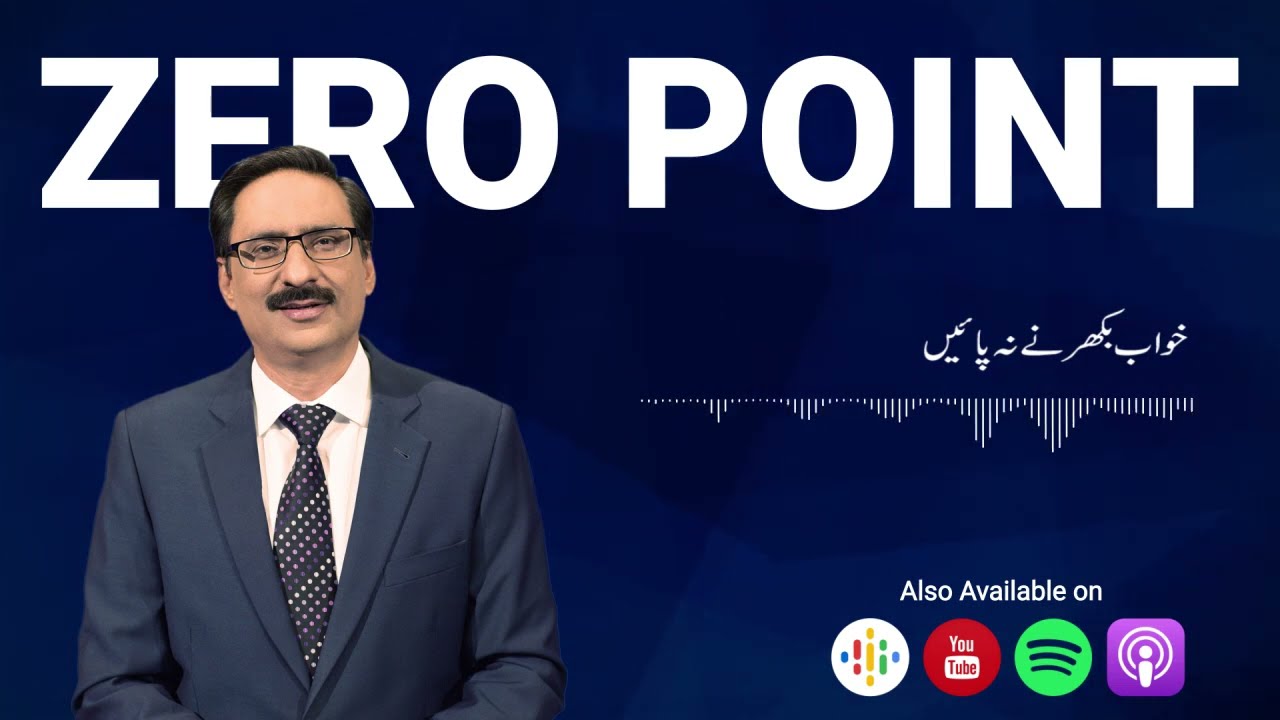This is a promotional image for a podcast or news show called "Zero Point." The image features a dark blue background divided into four slightly varying shades, creating a squarish corner pattern. At the top of the image, large, bold, white text reads "ZERO POINT." Positioned on the left is a man with short black hair, a thick mustache, and glasses, who is wearing a gray blazer over a white dress shirt and a tie with white, blue, and gray dots. This man looks directly at the camera. To his right, there are stylized inverted bar graphs resembling decibel measurements, situated below white text in a foreign language, likely Arabic or Indian. At the bottom right corner, white text states, "Also Available On," followed by a series of icons for platforms including YouTube (a red circle), Spotify (a green circle with three horizontal lines), and another platform represented by a purple square with a microphone and circles around it.